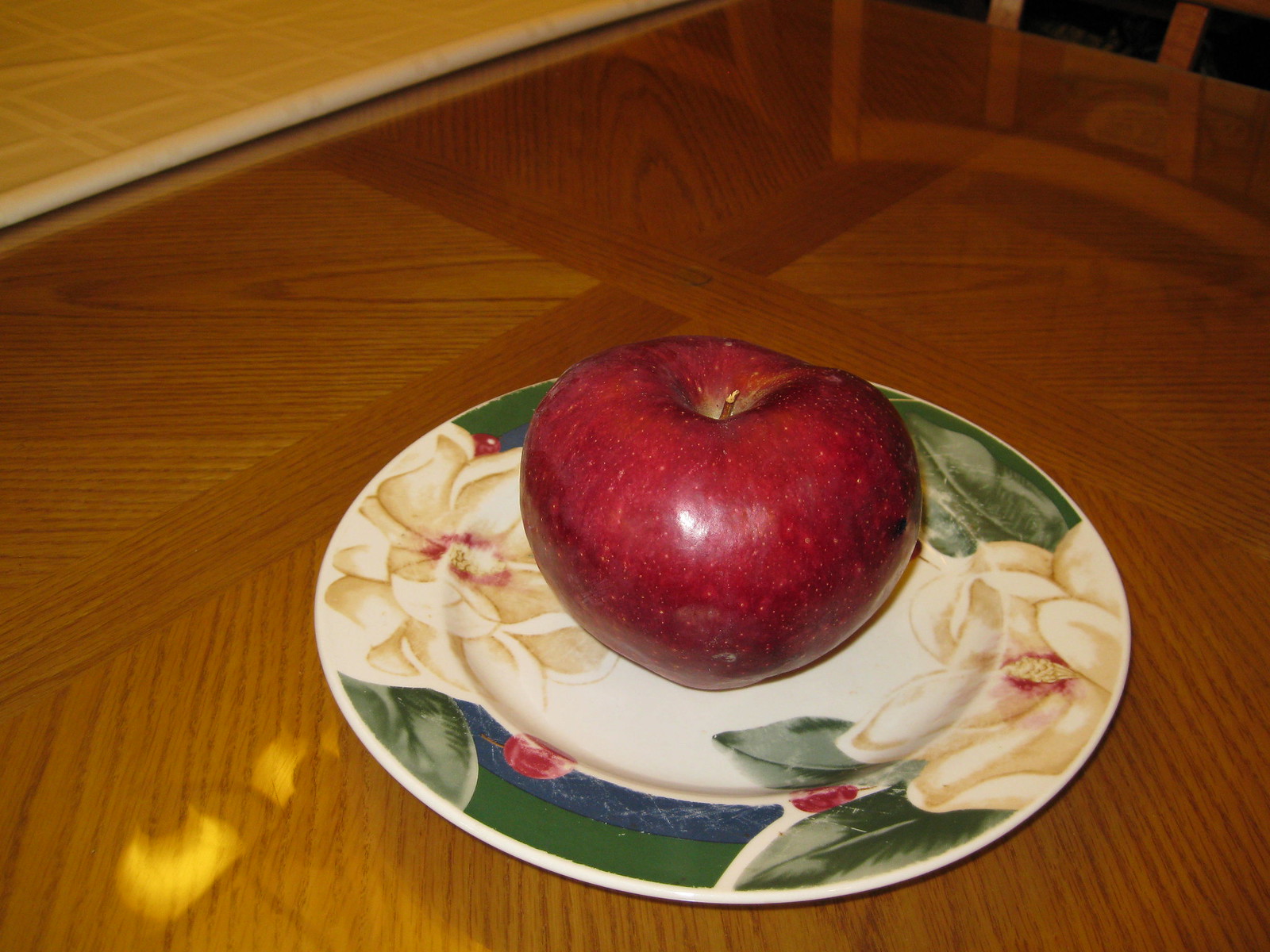The photograph is rectangular, with its longer sides at the top and bottom. At the center of the image, a single red apple takes focal prominence, its glossy skin highlighted against the backdrop. A brown stem protrudes from the top of the apple, adding a touch of natural imperfection. The apple rests on a solitary round porcelain plate. This plate is predominantly white, adorned with elegant floral designs around its rim, featuring two white flowers each on the left and right sides.

The plate is set upon a light brown, polished wooden table, composed of various square and rectangular wooden pieces with varying shades, from darker to lighter hues, creating a visually intriguing pattern. In the top left corner of the photo, a yellow fabric table runner with a subtle grid-like pattern adds warmth and contrast to the scene. The top right corner reveals the edge of a matching wooden chair, partially framing the image and adding depth, as the area behind the chair fades into an indistinct, shadowy black background. In the bottom left corner, the table’s surface reflects light from an overhead chandelier, lending a sparkle to this serene and meticulously arranged composition.